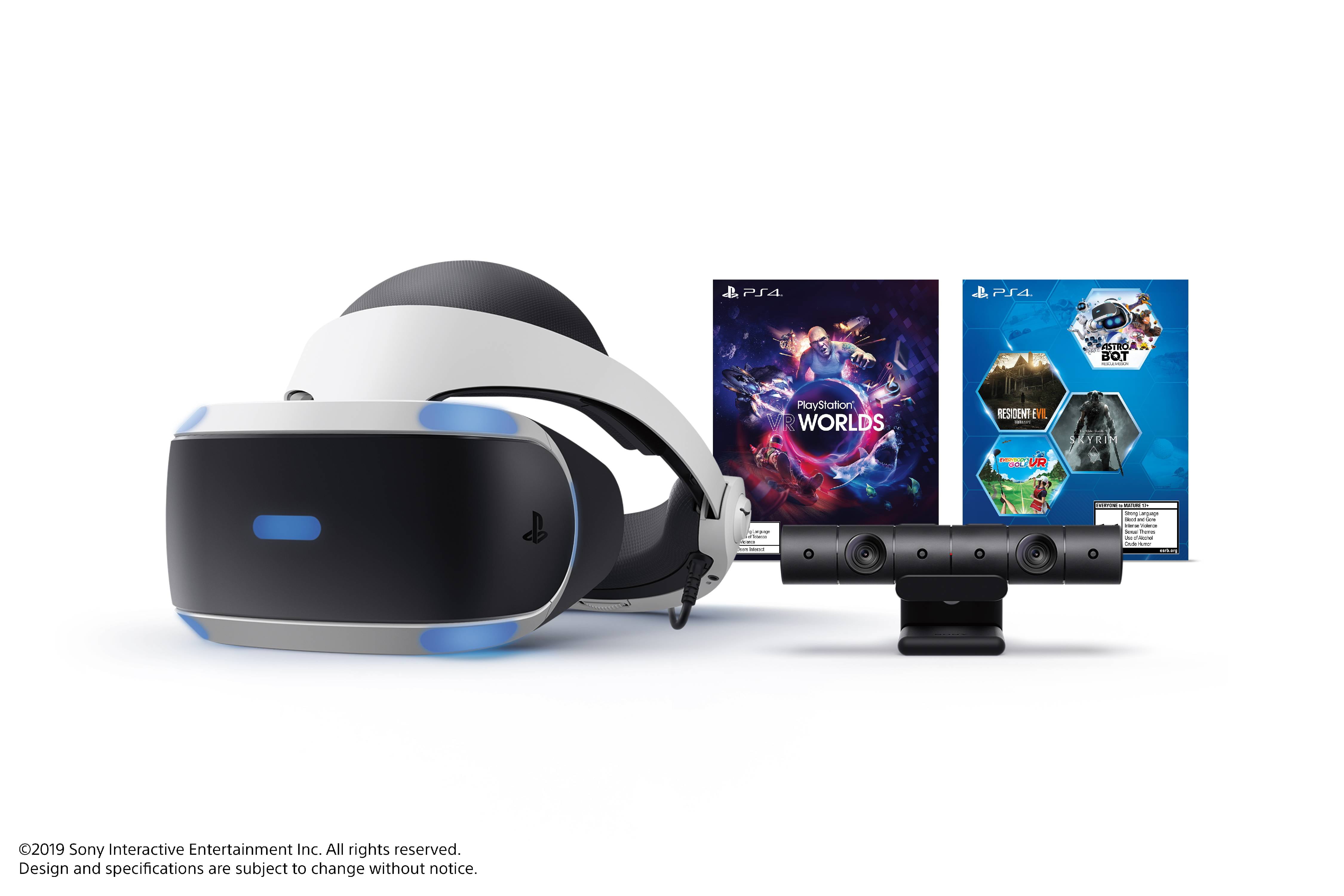This color photograph is a product image that prominently features a sleek VR headset on the left, and to its right, two PlayStation 4 game cases. The VR headset boasts a modern design with a predominantly black body accented by a silver metallic finish and a white adjustable strap that wraps around like a belt. To the right of the headset are two game cases, both displaying the PS4 logo in the upper left corner.

The game case on the left is predominantly black with pink and purple hues, featuring the title "PlayStation VR Worlds" in large white text and a person on the cover. The game case on the right has a blue background, showcasing various six-sided figures with unreadable text due to the small font size. The image background is a clean, solid white, emphasizing the products. 

In the lower left corner of the image, fine black print reads, "Copyright 2019, Sony Interactive Entertainment Incorporated. All rights reserved. Design and specifications are subject to change without notice."